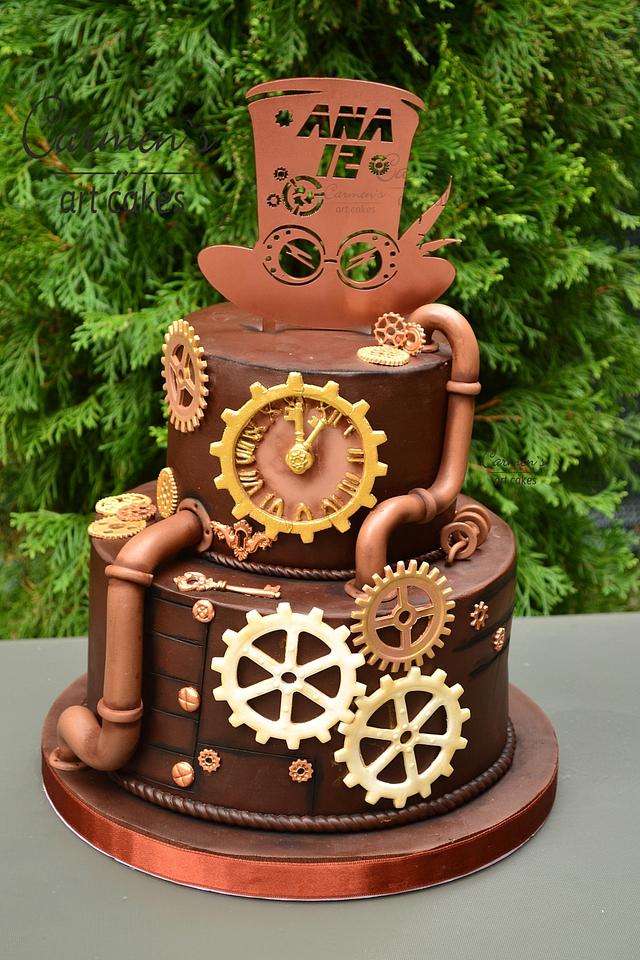This photograph captures an elaborate, custom-made steampunk-themed cake against a backdrop of lush green tree leaves. The cake rests on a brass-looking base placed on a gray table. The cake features two tiers adorned with intricate chocolate brown icing, meticulously designed to resemble metal. Atop the second layer sits a top hat with the inscription "ANA 12," hinting at a birthday celebration. Near the brim of the hat, fondant glasses add a whimsical touch. 

The second tier showcases a yellow clock with Roman numerals set at one o'clock, framed by a border of yellow gears. Additional gears and pipes, crafted from icing and fondant, interlock and wind around both layers of the cake, enhancing its mechanical aesthetic. Notable details include three interlocking gears on the lower tier in shades of yellow, white, cream, and brown, as well as smaller button gears and an old-fashioned key placed on the first layer.

The entire cake, though not gigantic, exudes a high level of craftsmanship and creativity, making it a fitting centerpiece for any themed celebration.